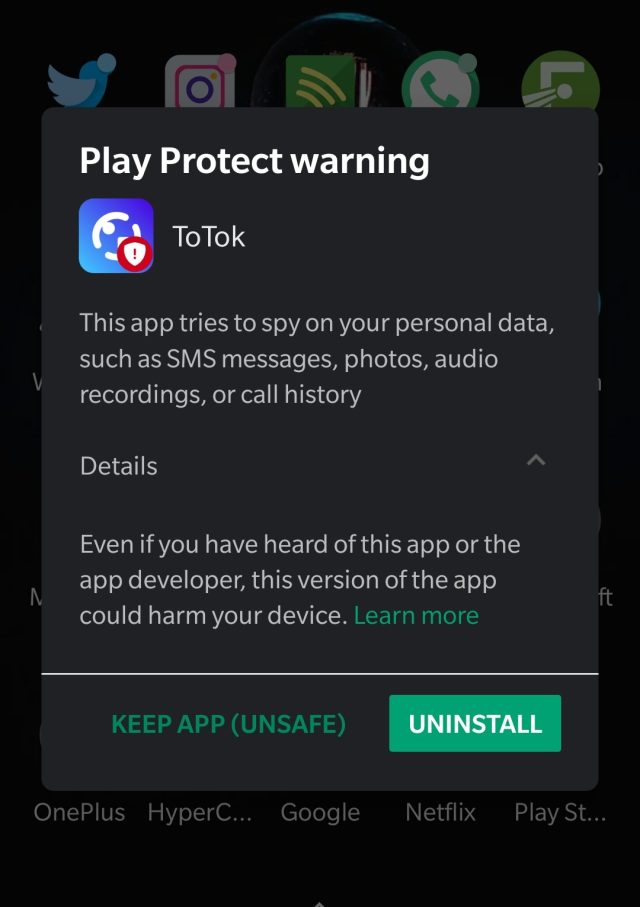The image depicts an overlay notification from Play Protect at the top of a device's home screen. The notification reads "PLAY PROTECT WARNING" in bold white lettering. Below this, there's an icon resembling a circle with a diagonal line through it, also in bold white.

The background transitions from dark blue in the upper right corner to light blue in the bottom left. On the overlay, there is a red caution symbol featuring a white shield with a red exclamation point. To the right of this symbol, the text "T O T O K" is written in white lettering with both T's capitalized.

In smaller light gray lettering, the notification states: "This app tries to spy on your personal data, such as SMS messages, photos, audio recordings, or call history." Followed by this, it reads: "DETAILS," then continues, "Even if you have heard of this app or the app developer, this version of the app could harm your device."

Below this text, the phrase "Learn more" is presented in green, suggesting it is clickable. There is a light gray or white divider line beneath this section, separating it from the following buttons: on the left, "KEEP APP (UNSAFE)" in bold green lettering, and on the right, a light green rectangle with "UNINSTALL" in capital white letters.

The background of the image displays a home screen with several app icons. The Twitter icon is visible towards the top left, alongside the Instagram icon. Other icons include one that resembles a signal, likely for WiFi or data, a phone symbol, and another symbol that appears to be a digital 'C' with two diagonal stripes and a ball at the end.